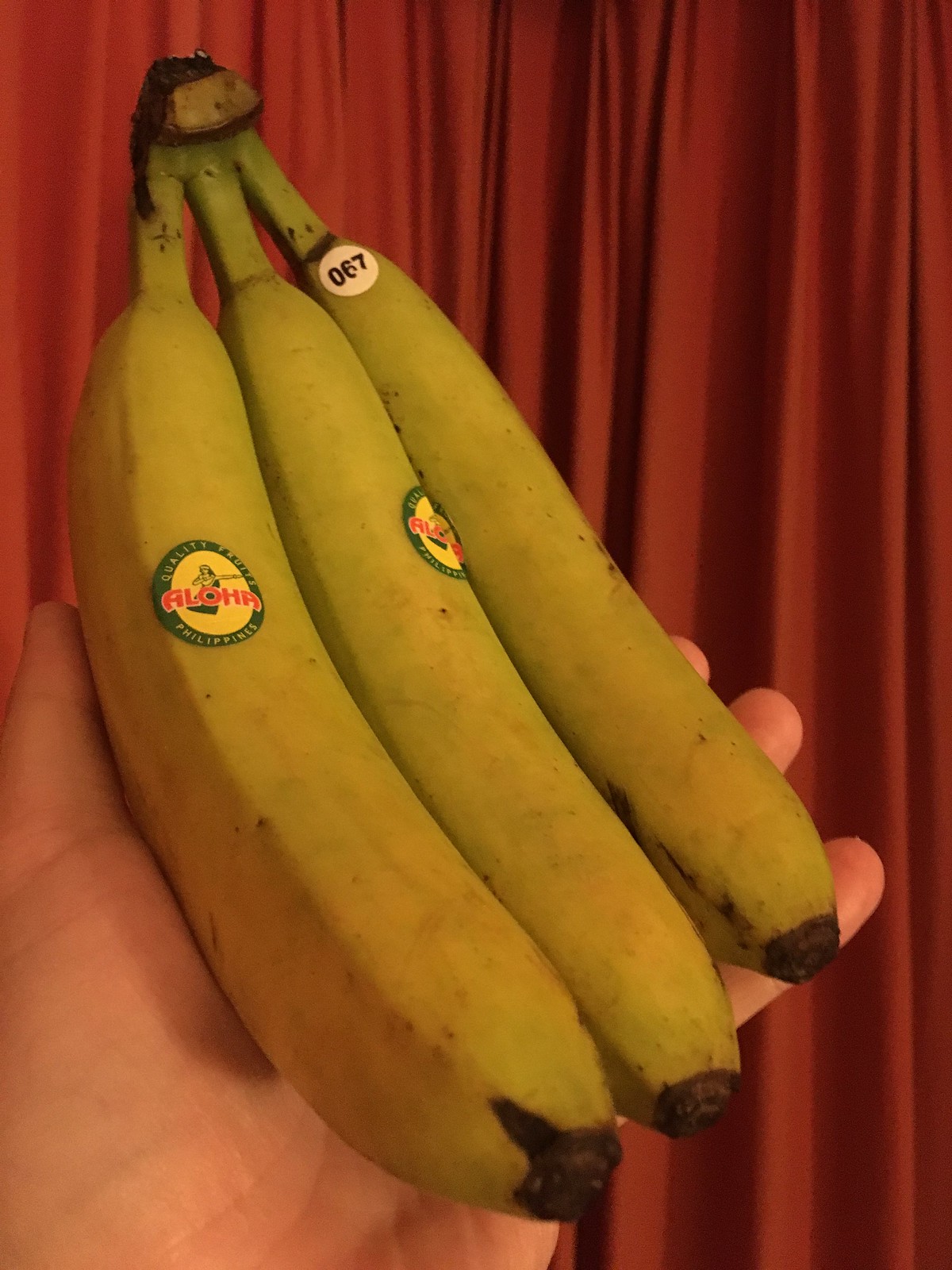In the foreground of the photograph, a pale-skinned hand with visible palm wrinkles and outstretched fingers is holding a bunch of three large, greenish-yellow bananas. Each banana is attached to a brown stem, and they exhibit no brown spots, indicating they are not fully ripe. The left and middle bananas each have a yellow and green sticker with the word "Aloha" in red capital letters, possibly showing a female hula dancer. The rightmost banana features a white sticker displaying the number "067." Dominating the background is a deeply ruffled, rust-colored curtain, which adds a rich, textured backdrop to the composition.